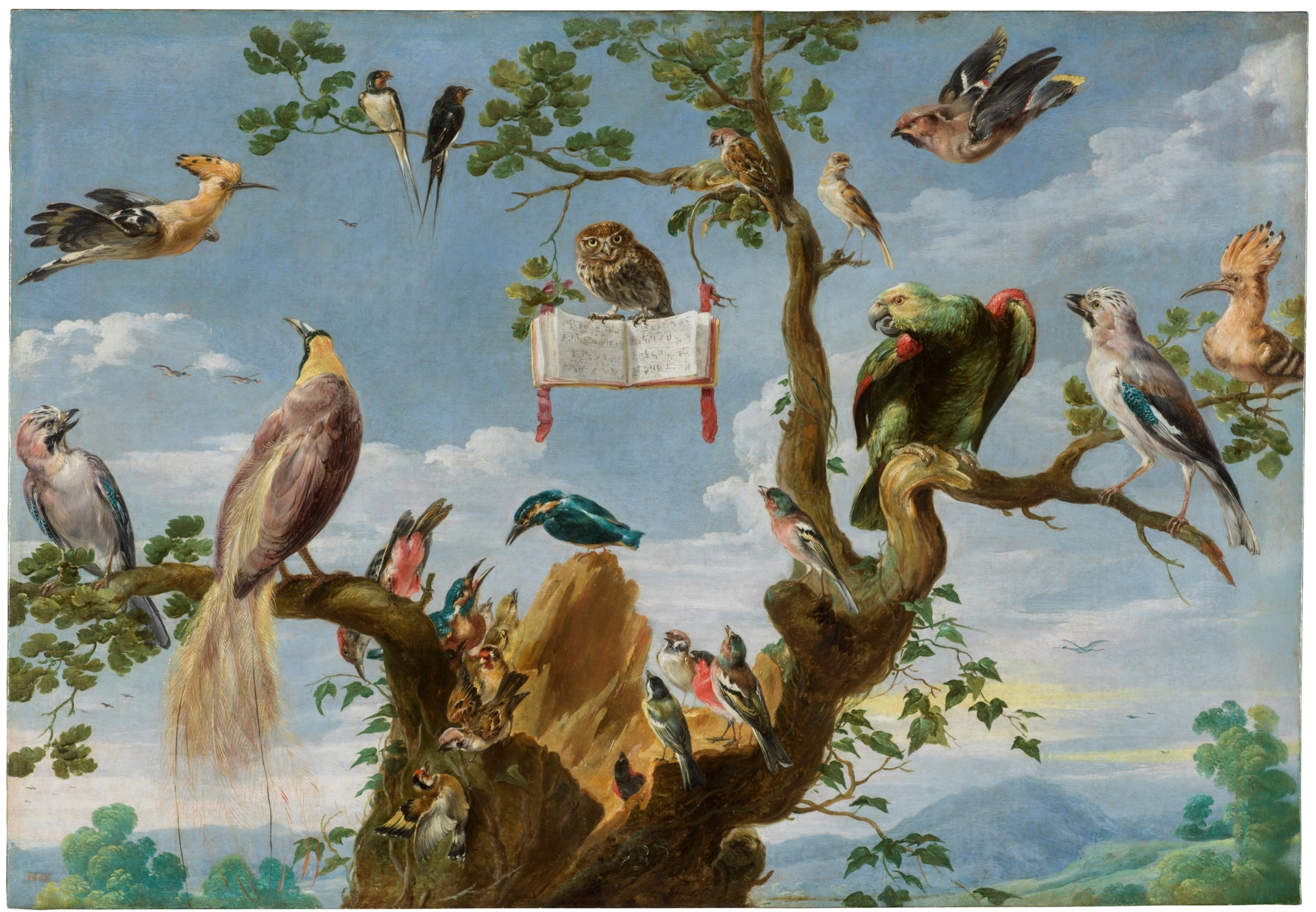In this detailed and intricately painted image, we see a vibrant array of birds perched atop a partially broken tree. The tree, which splits into three main branches, hosts a myriad of bird species, each varying in size, color, and type. Among the birds are owls, vultures, finches, robins, and a striking black bird with a yellow stripe on its head. The birds exhibit a rich palette, featuring grays, blues, reds, yellows, greens, and browns. 

At the heart of the painting, the central branch curves upward, adorned with smaller branches and leaves. These branches support an open book with dark gray writing, likely symbolic, as it is indistinct. The book, red in color and accented with red tassels on both sides, serves as a prominent focal point. Notably, an owl perches directly on this book. 

Some birds are depicted in flight—one on the left and another swooping down from the top right—adding dynamic movement to the scene. The background features a blue sky with white clouds, and distant trees, enhancing the depth of the landscape. This mural-like illustration, suggestive of an Audubon Society rendering, captures the diverse and vivid beauty of avian life in a detailed and elegantly painted tableau.